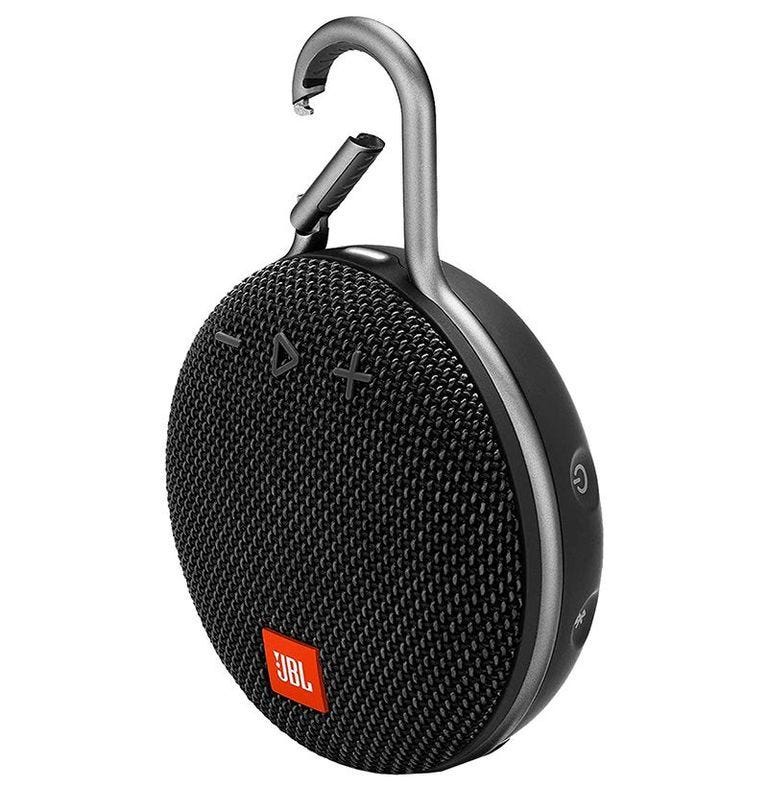This image features a sleek, modern wireless JBL speaker displayed against a white background. The speaker has a round, black body with a dimpled texture on the front. Prominently displayed on the front is a red logo with the brand name "JBL" in white letters. Situated at the top of the speaker’s front side are three symbols: a minus sign, a play symbol, and a plus sign, which allow you to easily control the volume and playback. On the right side, you can spot a gray power button. The speaker showcases two distinct textures: a dimpled front and a smoother back and side. A noteworthy feature is the silver metal carabiner clip at the top, which is open and allows you to attach the speaker to a belt or bag for convenience on the go.